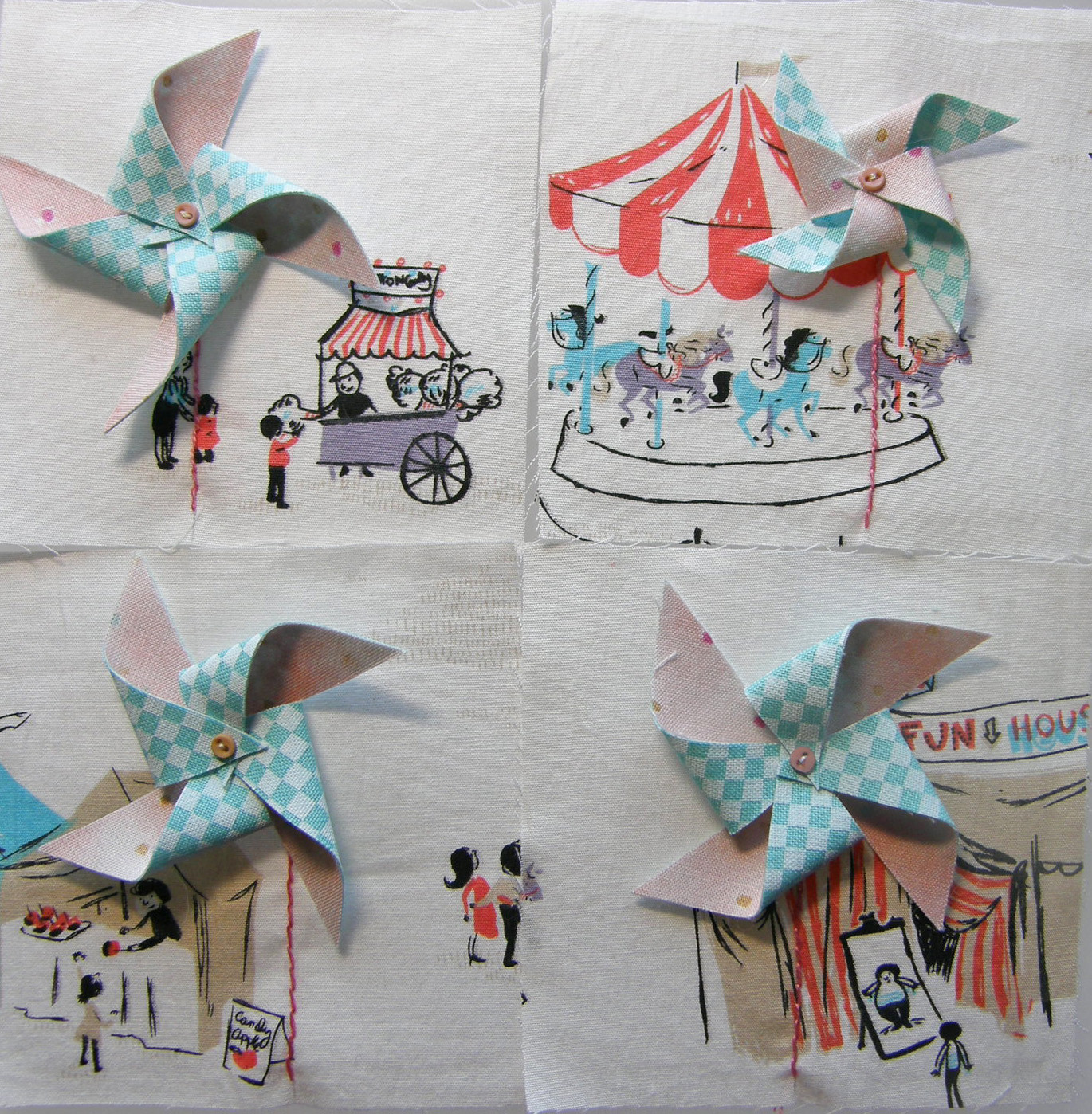The image consists of four whimsical, handcrafted fabric squares arranged in a two-by-two grid on a white background, each adorned with a central pinwheel made from blue and white checked fabric. Each square captures a lively carnival scene:

1. **Top Left**: A tiny handmade windmill pinwheel stands out against a pink backdrop, depicting a fair scene. Behind the windmill, there's a cotton candy stand with red and white striped roofing and a purple base with a single wheel. Two children in red shirts and an adult are buying cotton candy from a vendor in a black shirt and hat.

2. **Top Right**: Another pinwheel is part of a merry-go-round scene, featuring a red and white striped roof. The carousel is adorned with purple and blue horses, enhancing the festive atmosphere.

3. **Bottom Left**: This square includes a windmill pinwheel set against a scene with a woman in a red dress and a stand selling candied apples. The stand, manned by a person in black and accompanied by a girl in a gray dress, adds a sweet touch to the fairground depiction.

4. **Bottom Right**: The final square showcases a Funhouse indicated by a sign with red and gray curtains. Another pinwheel is placed nearby. A visitor stands in front of a funhouse mirror, appearing much larger in the reflection, adding a whimsical and humorous element.

The consistent use of blue and white pinwheels ties the images together, creating a cohesive and charming representation of a bustling carnival.